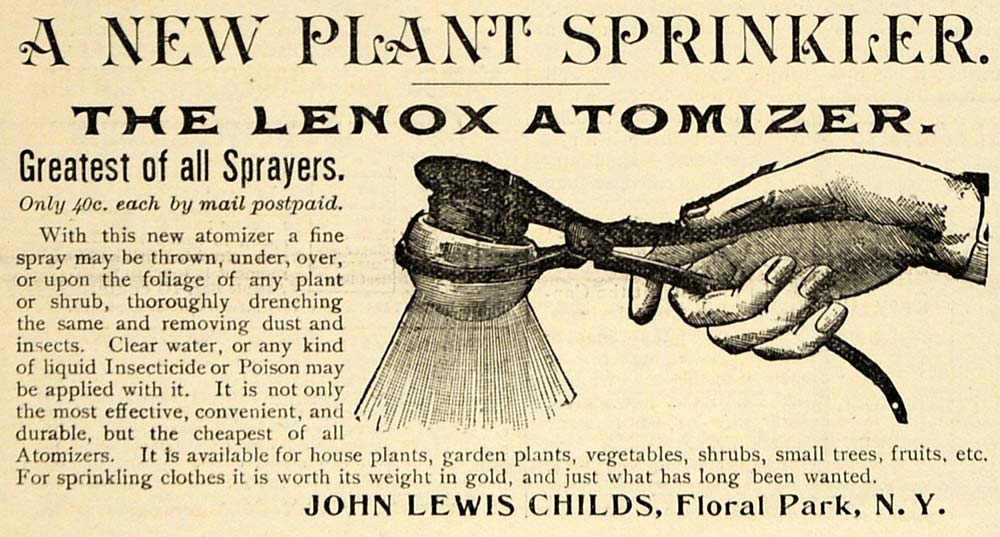This image features an historic advertisement set on a beige background with vintage black font. At the top, it announces "A New Plant Sprinkler, The Lennox Atomizer," proclaimed as the "Greatest of All Sprayers." The advertisement includes a detailed line drawing of the device, showing a hand holding a two-handled object attached to a hose, which emits a neat, uniform spray. The ad highlights that this innovative atomizer is priced at only 40 cents each, mail postpaid, emphasizing its affordability and era. A descriptive paragraph explains the atomizer's functionality, stating it can throw a fine spray under, over, or upon any plant or shrub, making it effective in removing dust and insects with water, insecticides, or other liquids. It extols the atomizer's convenience, durability, and cost-effectiveness, suitable for house plants, garden plants, vegetables, shrubs, small trees, and fruits, and even mentions its utility in sprinkling clothes. The bottom of the advertisement lists the name and location of the seller: John Lewis Childs of Floral Park, New York.